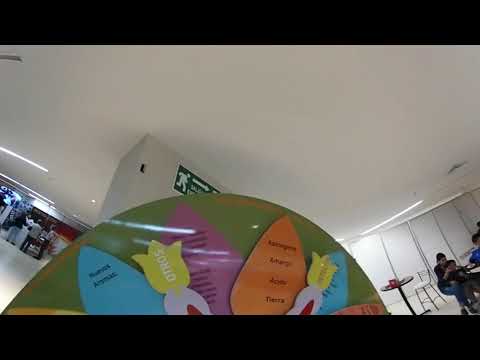The image captures the interior of a room with white walls and a high ceiling, shot from an upwards angle that causes a noticeable distortion, making objects appear misaligned. In the foreground, a large green semi-circular disc obscures much of the view. This disc resembles an arts and crafts project, adorned with multi-colored petal-shaped paper pieces—blue, orange, purple, and yellow—each with text on them, arranged to form a floral-like pattern. To the right, a seating area features tall black tables and white chairs, one of which is occupied by a mother with a child on her lap. To the left, another portion of the room reveals a counter with people standing and conversing in front of it, suggesting a possible storefront or cafe setting. The floor on either side of the image appears at unusual angles due to the distortion, adding to the overall disorienting effect.